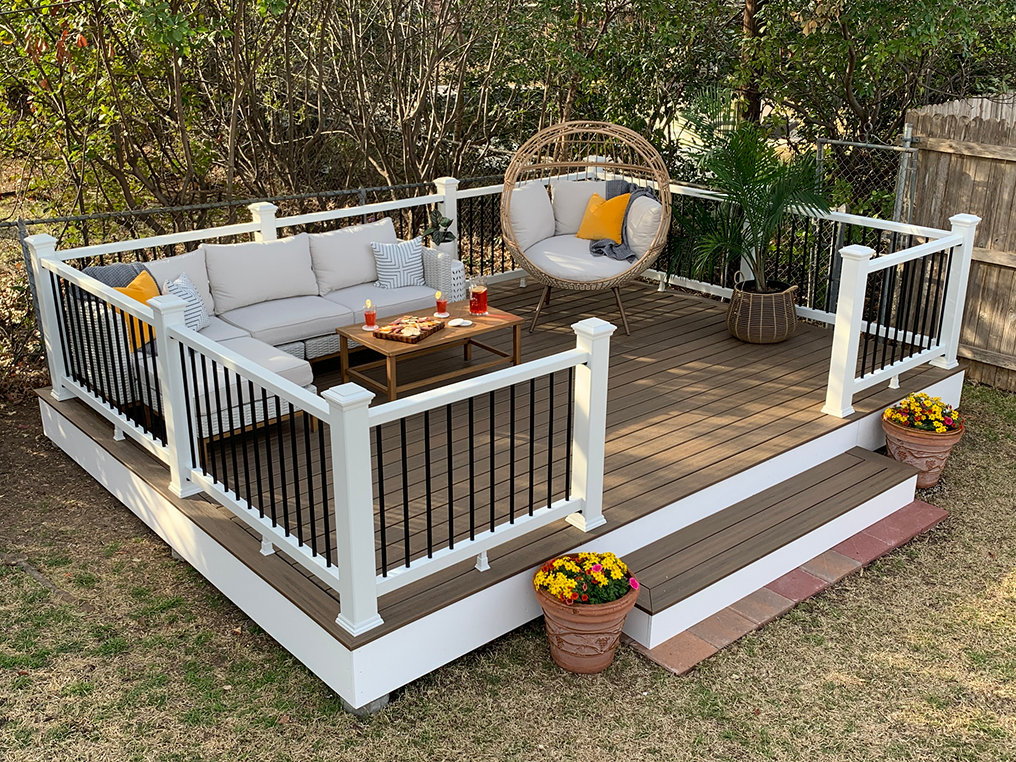This vibrant outdoor photo captures a meticulously staged backyard patio under a likely sunny sky. The square image, devoid of text, showcases a raised deck with a white wooden foundation and a stained hardwood floor. The deck is enclosed by a white post fence interspersed with black rails, except at the entrance, which has a single step leading down to brick-colored patio stones. Flanking the steps are terracotta pots blooming with red and yellow flowers. 

On the patio, an L-shaped sofa adorned with a mix of orange, gray, and off-white pillows stands as the main seating feature. In front of the sofa is a brown wooden coffee table holding a pitcher and glasses of iced tea along with some snacks. To the right of the coffee table is a large, cozy-looking wicker chair filled with multiple pillows in hues of off-white, gray, and orange. A wicker basket nearby also contains a plant, adding to the greenery of the setting.

The background reveals a chain link fence and some trees, with a wooden gate visible on the far upper right. The surrounding grass in the foreground appears dry and worn out. All elements, from the colorful pillows to the lush potted plants, contribute to a charming, inviting, and thoughtfully arranged outdoor space.